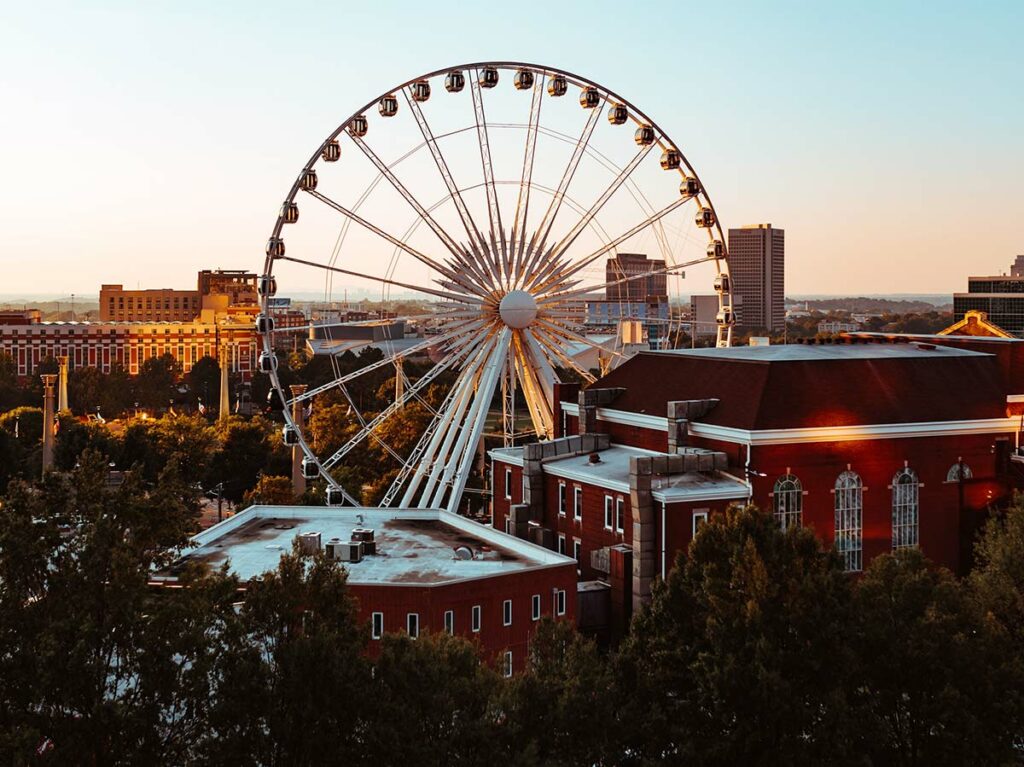The image captures a vibrant cityscape at either dusk or dawn, with a prominent Ferris wheel centrally positioned against a stunning backdrop. The Ferris wheel, with its white frame and enclosed cars, stands tall amidst an urban setting. Directly in front of it are two large red buildings, one appearing to be around two to three stories high with vertical windows reminiscent of stained glass, and the other slightly smaller yet similar in color and structure, adorned with small white windows on each floor. Both buildings suggest a purpose such as office space or perhaps a museum.

Surrounding the base of the Ferris wheel and the buildings, lush greenery with trees and bushes provides a natural contrast to the man-made structures. In the background, the skyline is dotted with a mix of architectural styles, including a flat-roofed, official-looking building to the left and a towering skyscraper to the right. The upper third of the image showcases a clear blue sky that deepens in hue from a pinkish horizon, contributing to the serene ambiance of the scene.